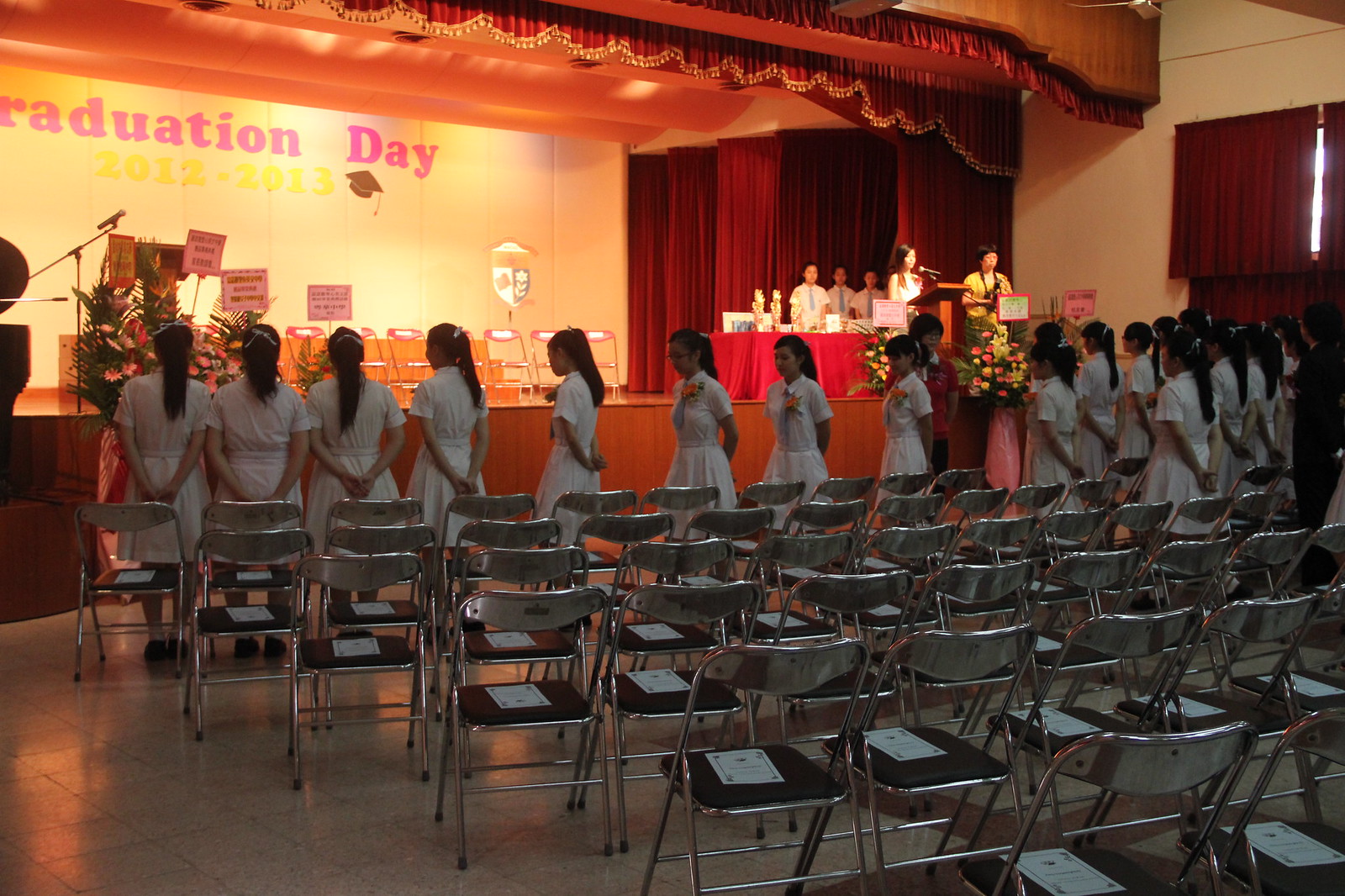The image captures a high school or college graduation ceremony set in an auditorium. The backdrop prominently displays "Graduation Day" in pink letters against an orange background, complemented by Chinese symbols and the drawing of a mortarboard. Rows of empty seats can be seen, except for a long line of approximately 25 to 30 young women in white dresses with corsages, wearing their long black hair tied back with white ribbons. They are approaching the stage, likely to take their seats or receive their diplomas. To the upper right of the photo, at a podium, a woman in a gold outfit is speaking. Behind her, three young men in blue ties and another woman holding a placard are positioned. The stage is further adorned with red curtains and a red tablecloth draped over a desk, adding to the ceremonious atmosphere. The overall scene is vibrant, capturing the essence of a significant milestone for these young women.